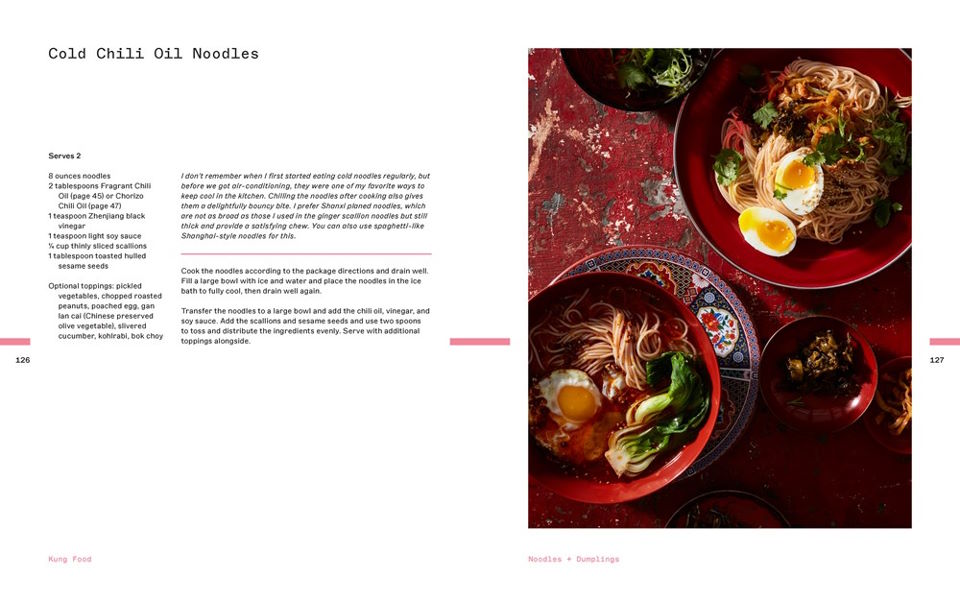Displayed in the image is a page torn from a cookbook, showcasing a detailed recipe for Cold Chili Oil Noodles against a white background. On the left-hand side, the recipe is clearly titled "Cold Chili Oil Noodles" followed by a comprehensive list of ingredients, which include eight ounces of noodles, two tablespoons of fragrant chili oil, one teaspoon of black vinegar, one teaspoon of light soy sauce, a quarter cup of thinly sliced scallions, and a tablespoon of toasted sesame seeds. However, part of the text is partially obscured and difficult to make out.

To the right, there's a vivid and colorful photograph of the completed dish, presented on an elaborate red, gray, and white Chinese tablecloth. The central focus is a red bowl placed on a matching plate, containing a serving of noodles topped with a sunny-side-up egg, onions, and garnished with green herbs, likely scallions. Beside it, there's a smaller bowl and an additional larger bowl showcasing medium-boiled eggs cut in half. Above, a black dish is also present, though its contents aren't clearly visible. The image portrays an elegant presentation with ingredients meticulously arranged alongside side dishes, demonstrating both the beauty and the intricate details of the meal.